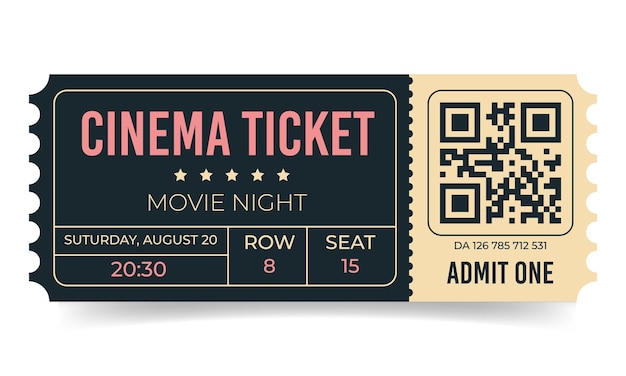The image is a close-up of a movie ticket set against a white background. The ticket itself is divided into two sections, with the left side being black and the right side tan. The edges of the ticket on both sides are ridged, indicating it has been perforated and torn. On the black side, the text "Cinema Ticket" is printed in red, followed by "Five Star Movie Night" in tan. Below this, it states the date, "Saturday, August 20," and the time, "2030." Further down, it specifies seating details: "Row 8" and "Seat 15." The tan-colored side features a prominently displayed QR code, with the text "Admit 1" located below it in black. Additionally, a number "DA 126 785 712 531" is printed beneath the QR code.